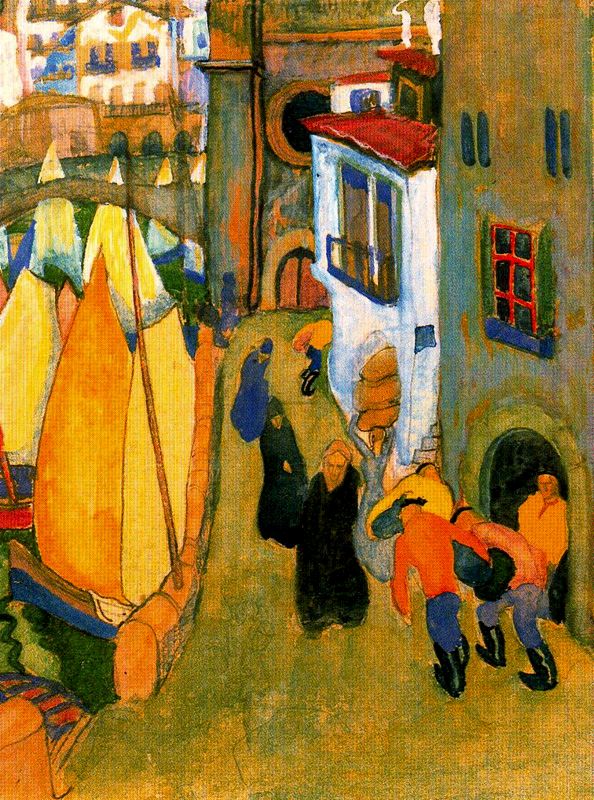This semi-impressionistic painting depicts a colorful, bustling street scene in a European village, likely from the 1500s or 1600s. Dominated by hues of green, orange, yellow, and splashes of blue and red, the scene is vibrant yet slightly surreal. On the right, a white building with a red rooftop and yellow-orange bordered windows stands prominently. The street, which appears to be going uphill, is lined with several buildings, including ones with olive-colored walls. 

Numerous figures dot the scene, adding to its lively nature. Six or seven people are visible, including two men in orange tops, black boots, and blue pants, looking down, possibly struggling with a black barrel. A woman in a blue gown confidently carries a load on her head, unfazed by the task, and is seen moving past the white building. Another woman in a long black coat walks nearby, adding to the diversity of the scene's characters.

To the left, sailboats with bright yellow and orange masts float on the water. The waterfront is bordered by curious yellow spiky tents or huts. The overall atmosphere is a juxtaposition of bright, cheerful colors and the rather somber, heavily clothed figures, creating an intriguing, almost timeless European street scene.